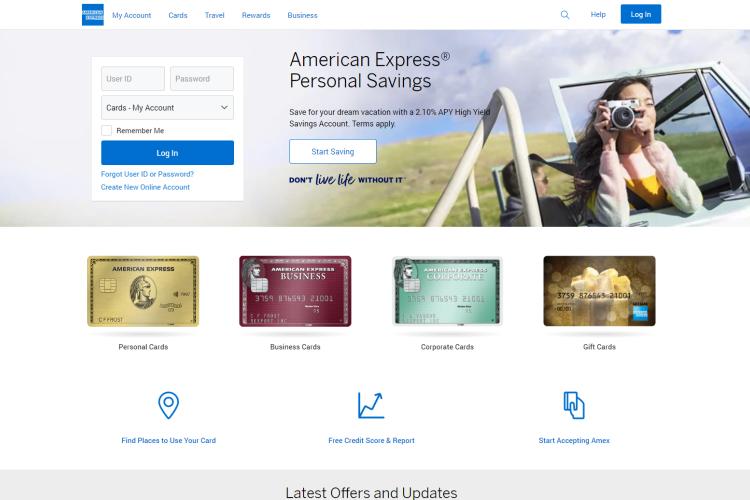The top section of the image features a white and blue background. At the center is the American Express logo, a white font within a blue square, though the text is slightly blurred. Adjacent to the logo, in white text on the blue background, are the navigation options: "My Account," "Cards," "Travel," "Rewards," "Business." To the right, there is a blue magnifying glass icon signaling the search function, alongside the word "Help". A blue rectangular button reads "Log In" in white text.

On the left-hand side, the background transitions to gray. It hosts various sign-in options and contains spaces to enter User ID and Password, both labeled in black text. Below, there’s a checkbox outlined in gray with black text next to it that says "Remember Me". A blue login button features white text saying "Log In". Underneath, blue text offers options such as "Forgot User ID or Password" and "Create New Online Account".

In black text, an advertisement encourages viewers to save for their dream vacation with a 2.10% APY High-Yield Savings Account, adding that terms apply. A blue text prompt reads "Start Saving" and a slogan "Don't Live Life Without It" follows in black. 

An adjacent image depicts a smiling female, holding up a camera and seemingly taking pictures as a male drives, suggesting a vacation scenario.

Below this, four card options are displayed. The first card is gold and labeled "Personal Cards", the second is burgundy marked "Business Cards", the third is green and says "Corporate Cards", and the fourth has a gold present icon and reads "Gift Cards".

Beneath these cards, blue text highlights various services, including "Find Places to Use Your Card", "Free Credit Scores and Reports", and "Start Accepting App Next". 

Lastly, the image concludes with a section in black text advertising "Later Offers" and "End Hour Updates".